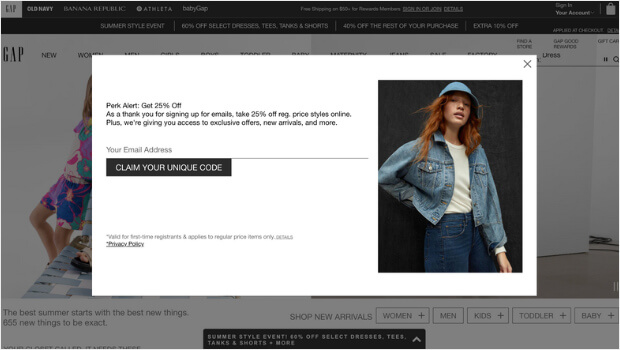The image features a screenshot of the GAP website with a promotional pop-up window overlaying the main content. The header of the website displays the names of associated brands: GAP, Old Navy, Banana Republic, Athleta, and Big GAP, with GAP being selected. Below the header, the main page showcases a woman dressed in summer attire consisting of shorts and a shirt, seated on what appears to be a summer lawn chair. The accompanying text highlights a seasonal promotion with the phrase, "The best summer starts with the best new things, 655 new things to be exact."

The pop-up window in the foreground depicts a woman wearing a jean jacket and a blue hat, with distinctive red hair. The pop-up includes a call-to-action button labeled "Claim Your Unique Code" and a text box for entering an email address, encouraging visitors with the message, "Perk Alert: Get 25% off."